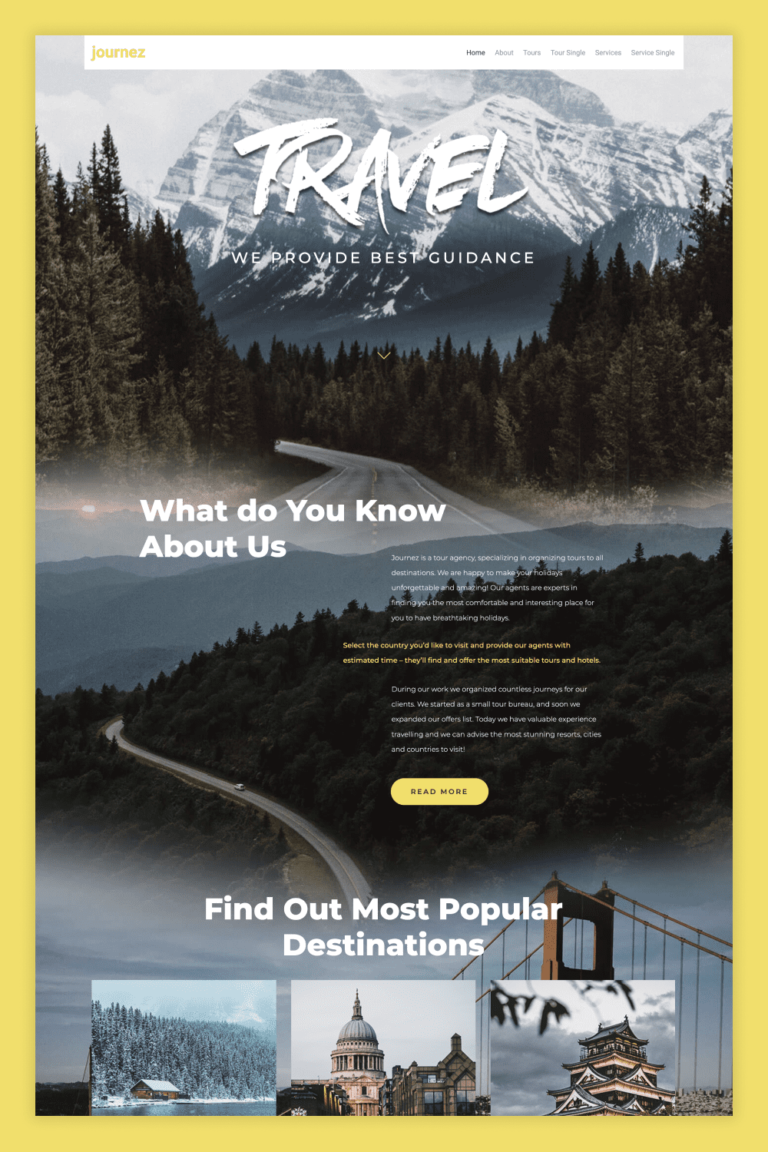The image resembles a magazine cover or perhaps a screenshot from a website, extending vertically in a long, continuous format that would span approximately three full desktop screens in height. 

The background prominently features a winding road that snakes its way through a lush, mountainous forest, flanked by majestic pine trees. As the eye travels upward, it reaches towering, snow-capped mountain peaks.

Overlaying the top portion of the image is a bold, white, scratchy font that appears as though it has been carved into stone, bearing the word "Travel." Below this title, in smaller white text, it reads, "We provide the best guidance." Further down, another line of white text questions, "What do you know about us?" Accompanying this text is a plethora of small, unreadable text, followed by a yellow "Read More" button inviting further exploration.

Enclosing the entire image is a yellow border, framing it elegantly like a picture.